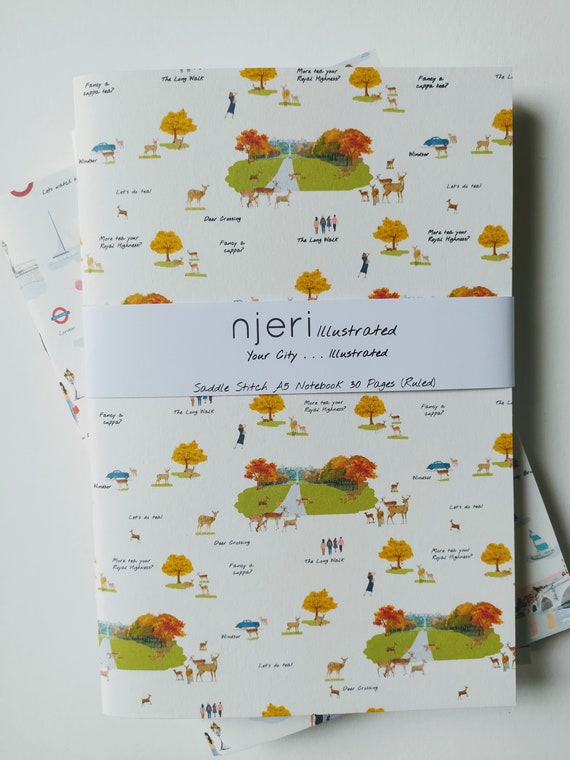The image features two thin, white notebooks, stacked one on top of the other, set against a plain white background. The top notebook is wrapped with a white ribbon bearing the text: "Ngeri Illustrated, Your City Illustrated, Saddle Stitch, A5 Notebook, 30 Pages, Ruled," indicating that it is a ruled notebook designed for writing. The cover of this notebook is adorned with a repetitive pattern of small illustrations, including trees, animals, green spots, and other elements of nature, suggesting a park-like theme. The second notebook, partially visible beneath the top one, shares the same white cover but lacks further distinguishable details.